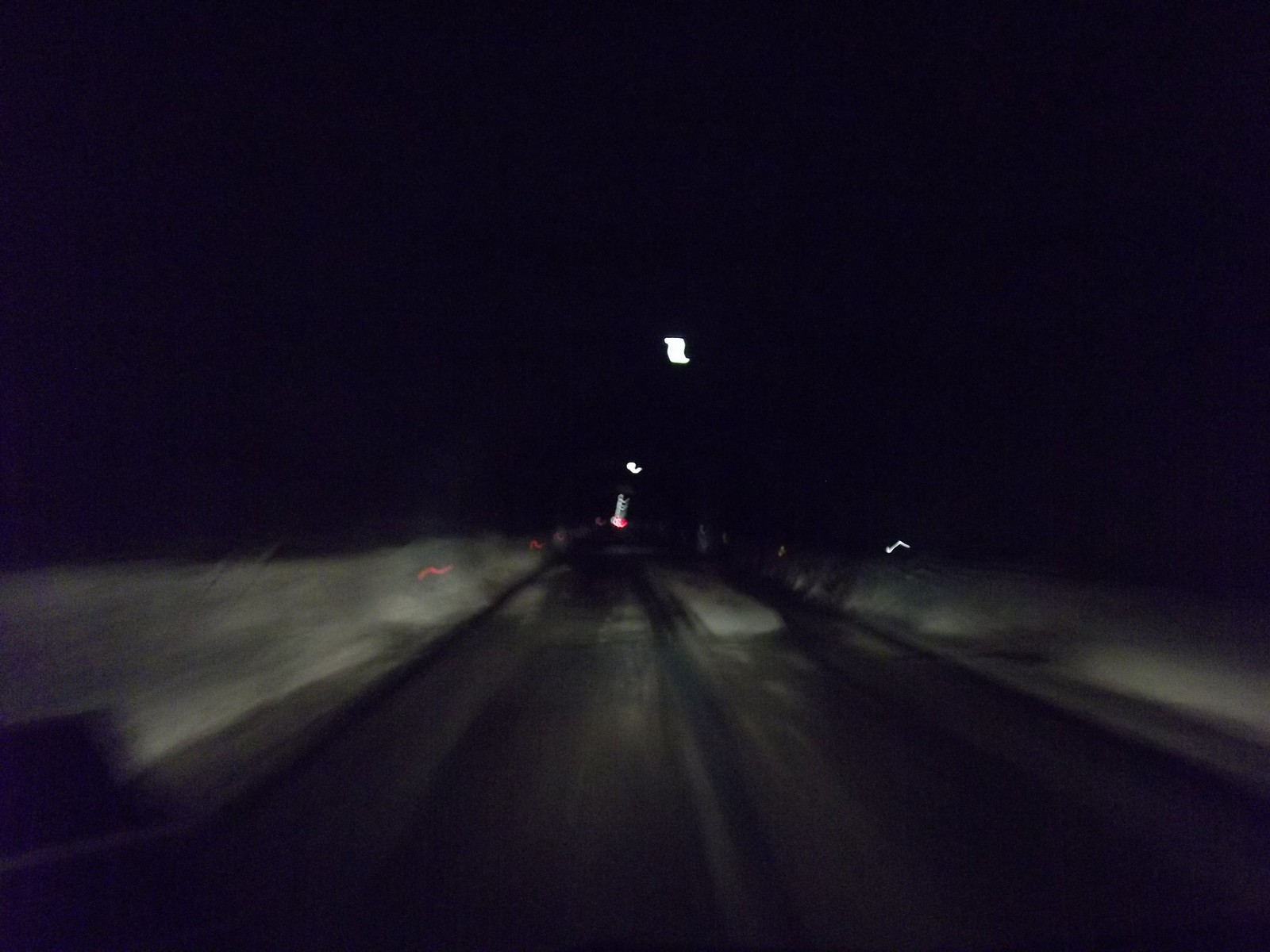This photograph, taken from inside a moving vehicle at night, captures a dark, dimly lit road shrouded in an eerie stillness. The sky above is pitch black, adding to the sense of isolation. A few scattered streetlights offer minimal illumination, spaced far apart on what looks like concrete sections at the road's edge. The road itself is layered with a mix of brown slush and accumulated snow, creating a textured surface that varies in color from dark black to lighter gray patches. Motion blur from the vehicle adds to the feeling of motion. Snow banks line both sides of the road, resembling thick, white blankets. In the distance, the faint red and white lights of other vehicles punctuate the darkness, while the vehicle's own headlights cut through the gloom, providing the primary source of light on the road. A peculiar, bright rectangular shape hovers in the sky, adding an element of mystery to the scene.